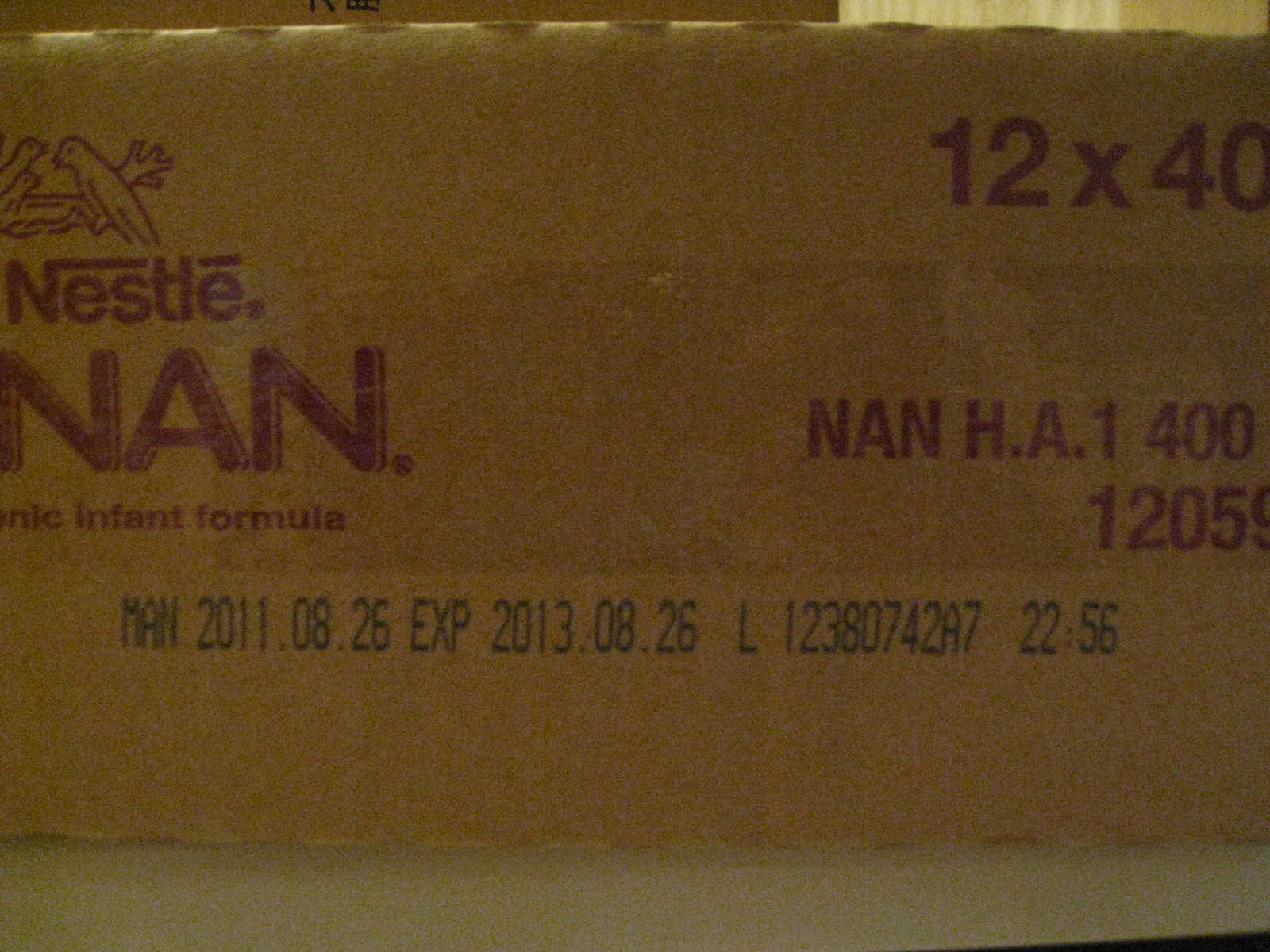The image features a piece of brown cardboard with various text markings and details. In the top left corner, the space is blank. Located on the middle left is the word “none.” The right section displays the phrase “ORGANIC INPUT FORMULA,” and the top right corner is marked with dimensions “12 x 40.” Directly beneath these dimensions, the word “none” appears again. There’s also a code that reads “H.A. 1400,” followed by the sequence “1205.” Below this, there are two dates: “MAN 2011.08.26” indicating the manufacturing date, and “EXP 2013.08.26” for the expiry date. Additional text “L 12387 074287” is present, along with the number “22.56.”

Furthermore, the box features dashed lines along the top and bottom edges. At the very bottom of the box, there appears to be a strip of white metal. The very top edge of the image shows part of the background of the room. Finally, there is a strip of tape extending from just above the word “none” on the left side, covering part of the text, and continuing towards the right end of the box.

This meticulous description captures all the textual and structural elements visible on the cardboard box in the image.